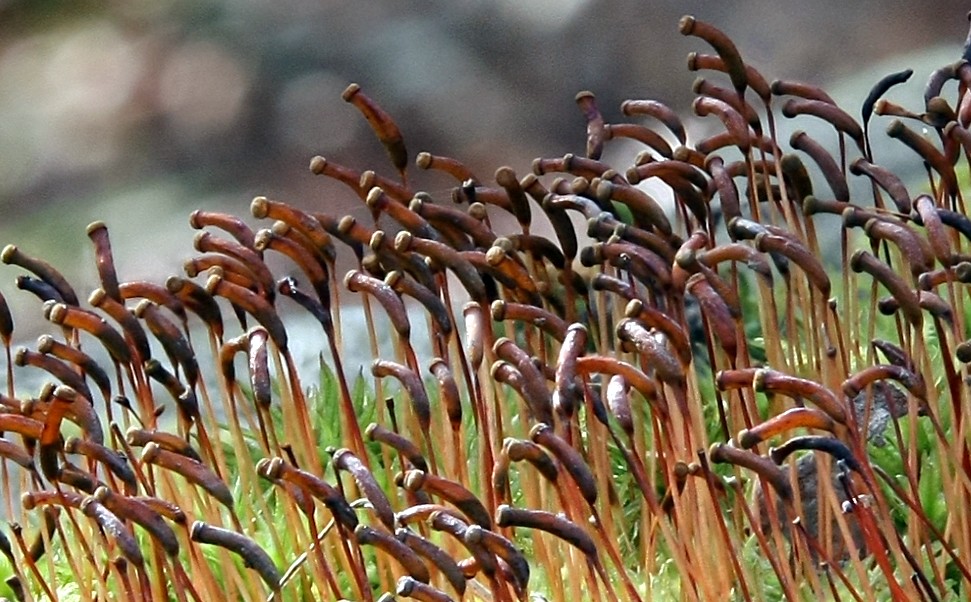The photograph captures a unique and peculiar field of Ceratodon purpureus, characterized by numerous stalks resembling a hybrid of human fingers and mushrooms. These tubular structures are all arching in a unified direction, primarily to the left, and display a range of brown, orange, and dark brown hues. Some parts of the stalks appear more dark orange, likely due to sunlight exposure. The stems are predominantly yellow, transitioning to darker shades, topped with knobs varying in darker tones. The scene is densely populated, with over a hundred of these stalks at differing heights, creating an undulating pattern across the field. The backdrop features a lush green carpet of grass, leaves, and other plants, fading into an out-of-focus area composed of blurry hexagon-shaped lights, enhancing the attention on the distinct foreground. The overall impression is one of an otherworldly or alien landscape, filled with these intriguing, finger-like plants.